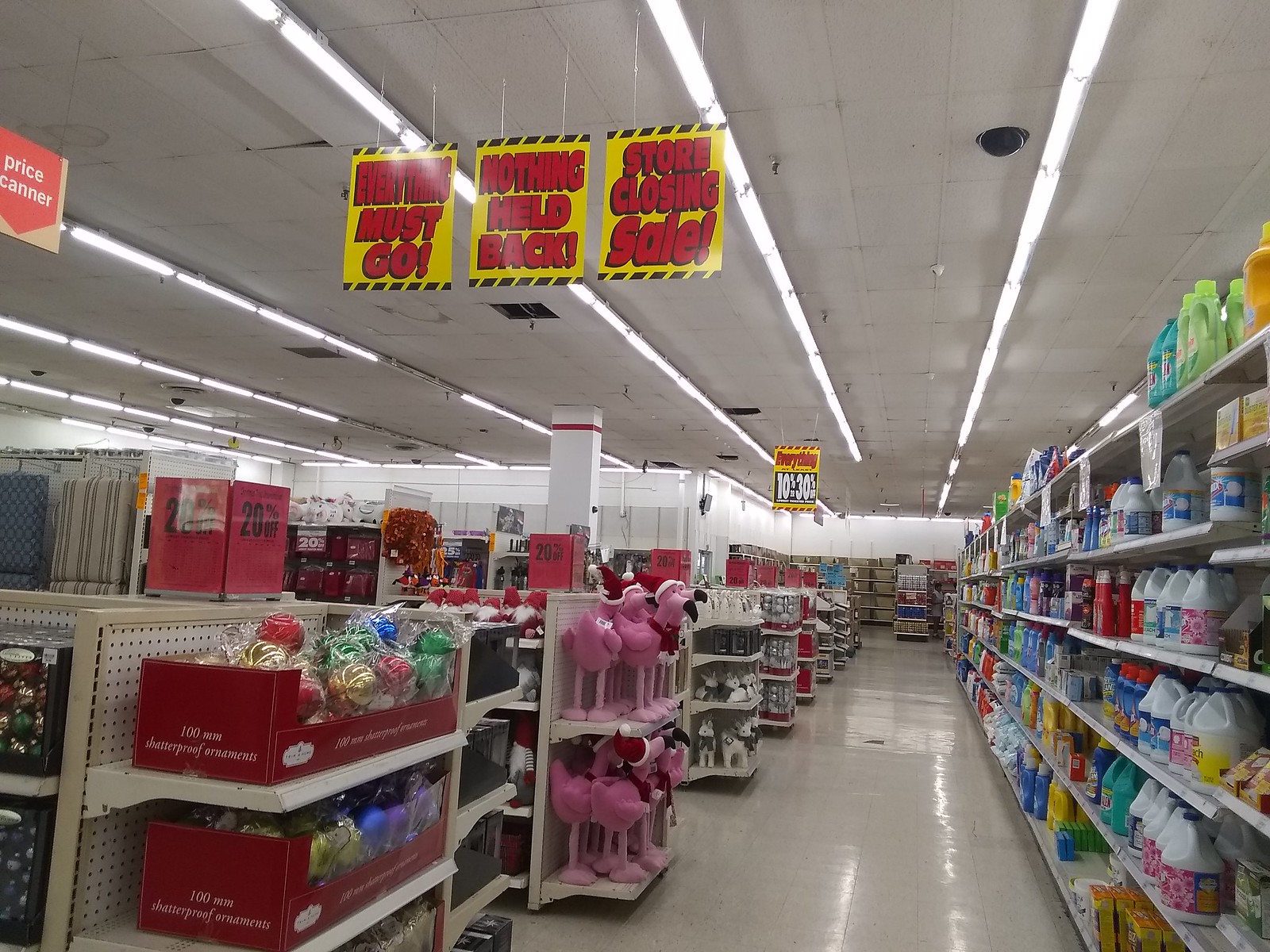This photograph appears to be taken inside a discount retail store, potentially a Dollar Tree or Family Dollar. The shot is captured from the back of the store, offering a view down the rear aisle. Shelves on both sides are fully stocked, including the aisle endcaps, which are decorated with various Christmas items. Notably, there are numerous pink flamingo ornaments dressed in Santa hats, adding a whimsical festive touch.

To the right along the back wall, shelves are lined with cleaning supplies such as bottles of bleach and mopping products. Prominent signs hang from the ceiling, displaying messages such as "Everything 10 to 30% Off," and "Everything Must Go," indicating that the store is undergoing a closing sale with no items being held back.